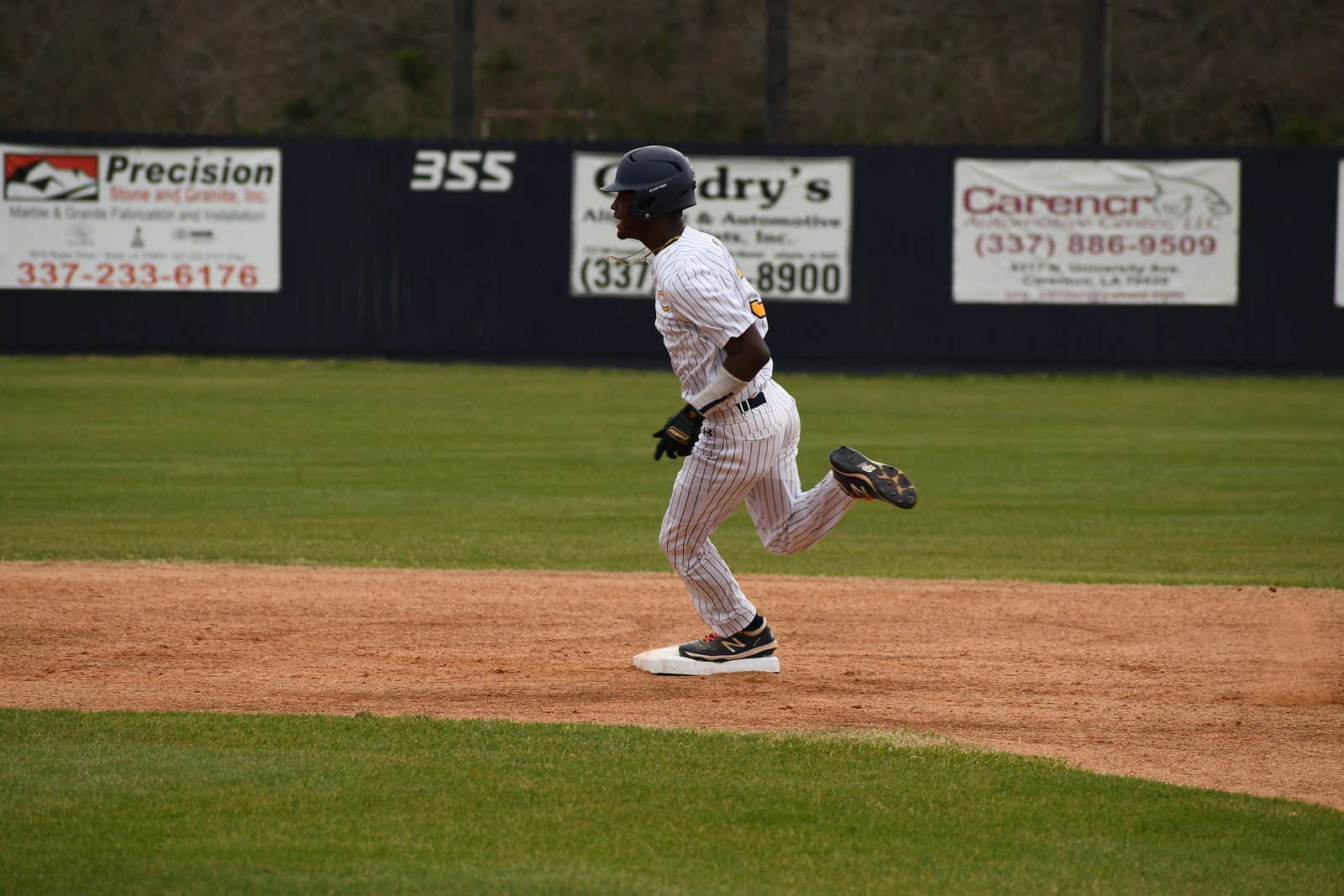The photograph captures a dynamic moment in a baseball game, featuring a black player in mid-stride as he runs the bases, positioned on one leg with the other raised and bent at the knee. Dressed in a white pinstripe uniform with black gloves, cleats, and a dark helmet, he stands out vividly against the lush green infield grass and the dirt base path. The background displays a dark-colored wall adorned with various advertisements, including a visible distance marker of 355 feet. The scene occurs outdoors on a cloudy day, adding an atmospheric touch to the action.